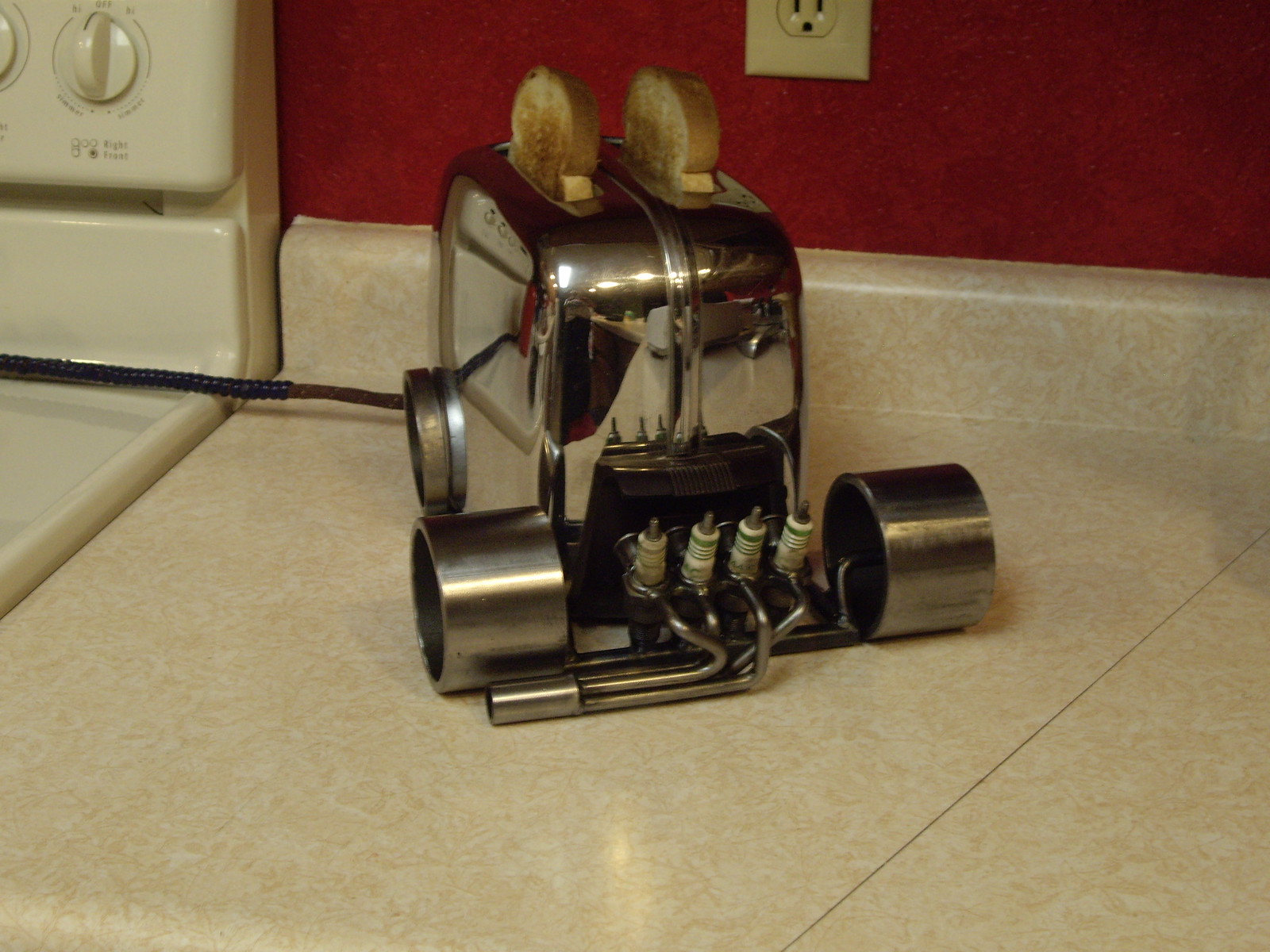This photograph depicts a highly polished chrome, two-slice toaster resting on a light tan, marbled-patterned countertop with a matching backsplash. The counter is situated in a kitchen setting, with a white stove visible to the left and a deep maroon-red wall behind it, featuring a cream-colored electrical outlet. The toaster is adorned in a 1930s, streamlined, antique style, and both slices of toast are visibly browned and popped up out of the slots. An intriguing mechanical contraption is attached to the front of the toaster, featuring four spark plug-like components with green rings, two large wheels on either side, and various metallic hoses, reminiscent of a miniature vehicle or a hot rod. A black power cord extends from the back of the toaster towards the stove. The image is detailed and realistic, with every element contributing to the vintage yet whimsical aesthetic of the scene.